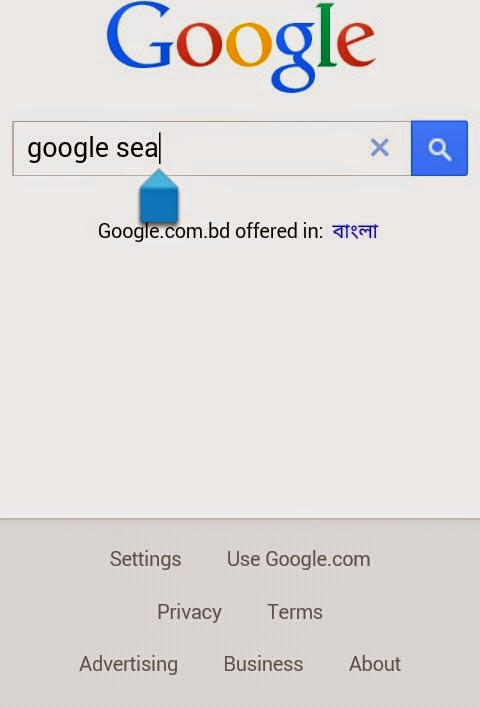Screenshot of a Google Search Page with SEA Query:

The screenshot captures the top portion of a Google search page. Dominating the top is the iconic Google logo, prominently displayed in its standard primary color scheme. The "G" is blue, followed by a red "o", a yellow "o", another blue "g", and finishing with "le" in red.

Directly beneath the logo is the Google search field containing the query "Google SEA" with an active cursor blinking to the right of the text. At the end of the search field are a small "x" button for clearing the input and a magnifying glass icon symbolizing the search function.

Below the search bar, in black font, the text reads "google.com.bd offered in:", followed by a script that appears to be an unfamiliar Southeast Asian language.

At the very bottom of the screenshot is a gray rectangle featuring clickable links, including "Settings", "Use Google.com", "Privacy", "Terms", "Advertising", "Business", and "About".

The entire screenshot is tinged with a gray filter, differing from the usual white background typical of Google's interface.